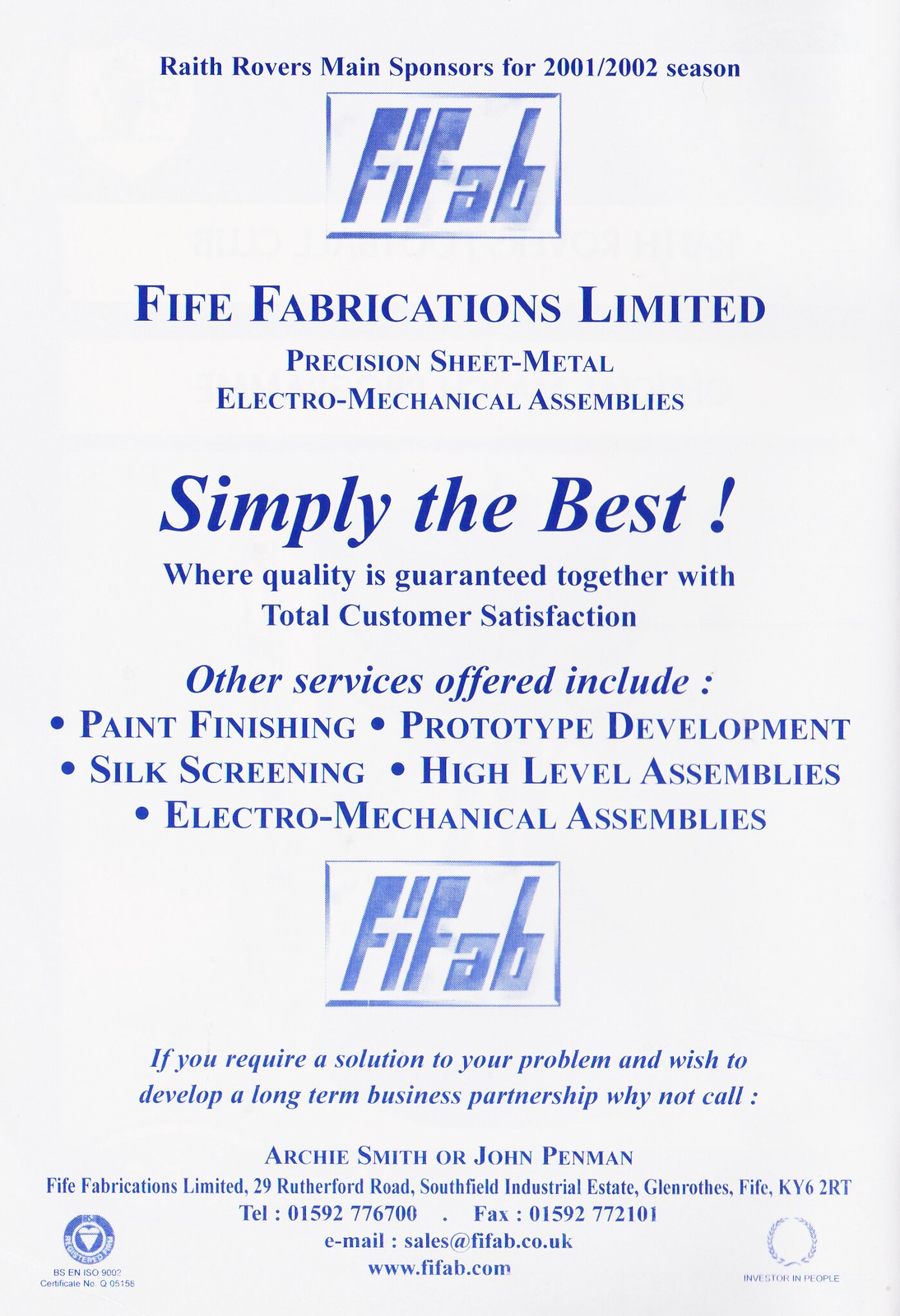This vertically aligned rectangular image, likely the cover of a booklet, features a light gray or white background adorned with blueprints. At the top, it prominently displays "Wraith Rovers Main Sponsors for the 2001-2002 Season." Below this header is a small rectangle with "FI FAB" inside, followed by the text "Fife Fabrications Limited" in bold, uppercase blue letters. This is immediately followed by the services offered: "Precision Sheet Metal Electromechanical Assemblies."

Midway down the cover, the phrase "Simply the Best!" in large blue text stands out, followed by the slogan "Where Quality is Guaranteed Together with Total Customer Satisfaction." Further down, the image lists additional services offered, complete with bullet points: Paint Finishing, Silk Screening, Electromechanical Assemblies, Prototype Development, and High-Level Assemblies.

Towards the bottom, the "FI FAB" logo reappears inside a blue-bordered rectangle. Below this, the text reads, "If you require a solution to your problem and wish to develop a long-term business partnership, why not call Archie Smith or John Pedman?" The address, phone number, and fax for Fife Fabrications Limited in Glenrothes, UK, are provided, along with the email address sales@fifefab.co.uk.